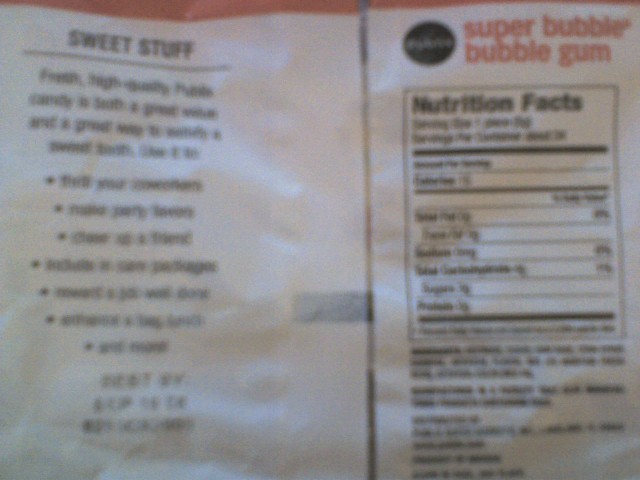The image depicts a very blurry back view of a product label, primarily featuring two main items on a red table. On the left, there's an advertisement labeled "Sweet Stuff," which has black text that's nearly impossible to decipher due to the blurriness. There's a hint of a potential "best by" date stamped at the bottom in black font, but it's too fuzzy to confirm. On the right side, we see a package with an orange section at the top reading "Super Bubble Bubble Gum" in pink text. Below this, there’s a black oval label with unreadable white text, followed by a nutrition facts box. Some details like "nutrition facts" and parts of the ingredients list can be faintly made out, while the rest of the text, including any further nutritional information and potential contact details, remains indistinct due to the heavy blurriness of the image.